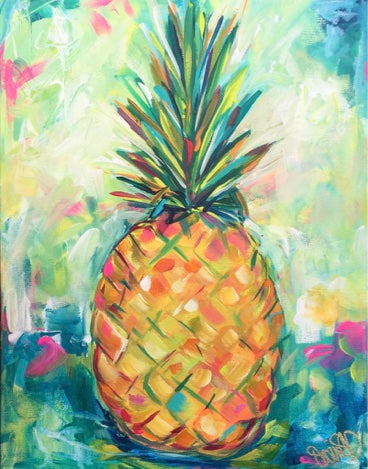This is an abstract, brightly colored watercolor painting of a single pineapple in a portrait layout. The pineapple itself features an explosion of colors, including shades of yellow, orange, pink, white, and even some blue. The leaves extending from the top showcase a mix of greens, blues, and yellows with touches of red. The background is a gradient of colors, with the upper left and right areas displaying lighter hues of greens, blues, pinks, and whites, and the bottom part showing darker green and blue tones along with some pinks. The setting appears to be a counter with a lighter wall behind it, further emphasizing the vibrant and unconventional color palette. The artist's signature is elegantly inscribed in gold in the lower right-hand corner. This artwork is not intended to be realistic but rather a creative and colorful representation of a pineapple.